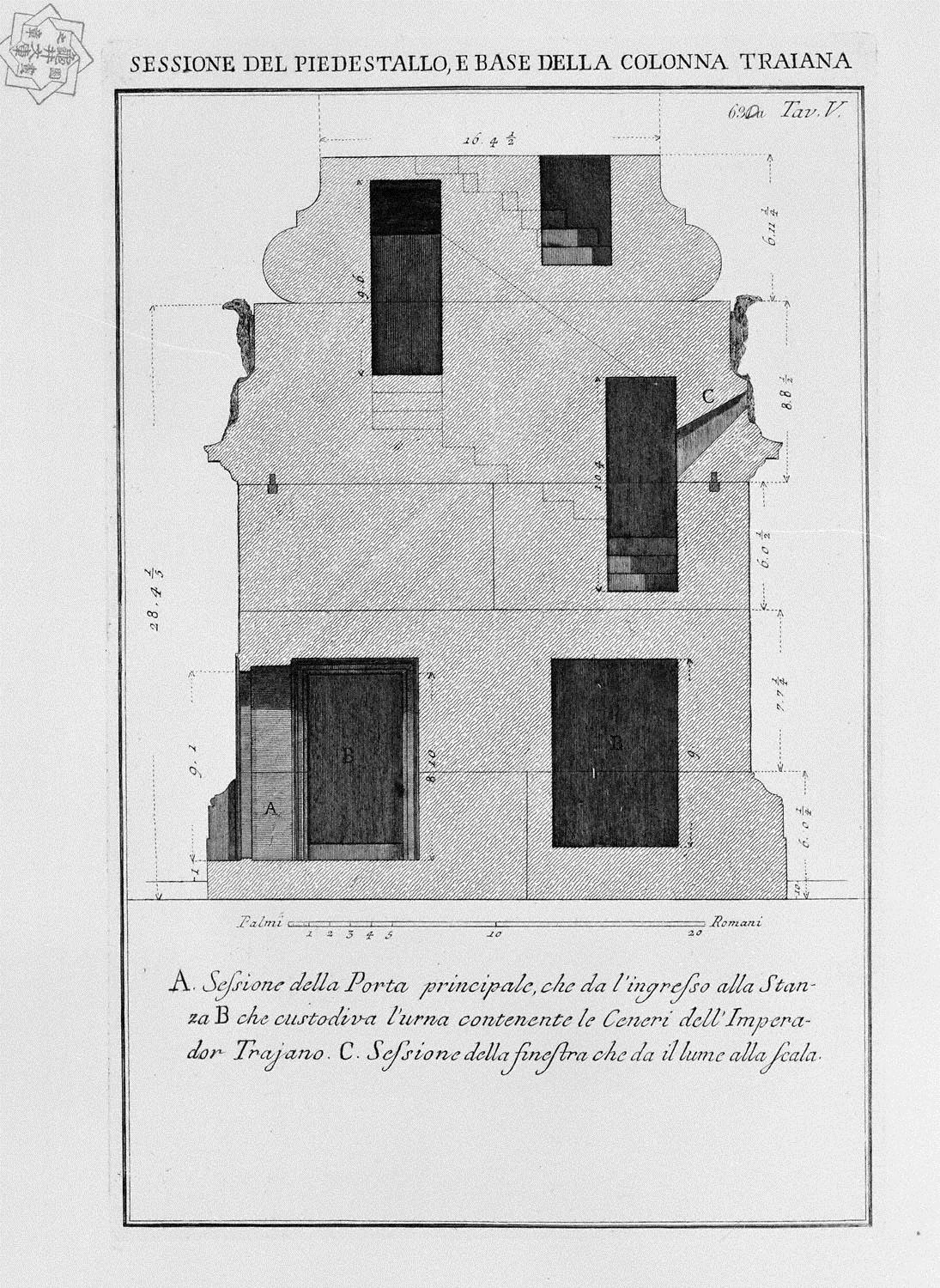The image appears to be an architectural blueprint or diagram in grayscale on a light blue background, bordered by a thin black line. At the top of the diagram, text reads "SESSIONE DEL PIEDESTALLO E BASE DELLA COLONNA TRAIANA," indicating it is written in Italian. The blueprint features a detailed side view of a three-story building, showcasing various architectural elements such as doors, windows, and staircases, marked by cutouts and measurements. The diagram includes rectangular display graphics and a stamp in the upper left-hand corner, suggesting authenticity or official approval. Below the detailed drawing, there is a paragraph of descriptive text in Italian, written in italics, which likely explains the various components of the building. Overall, the document appears to be a professional and intricate architectural representation.